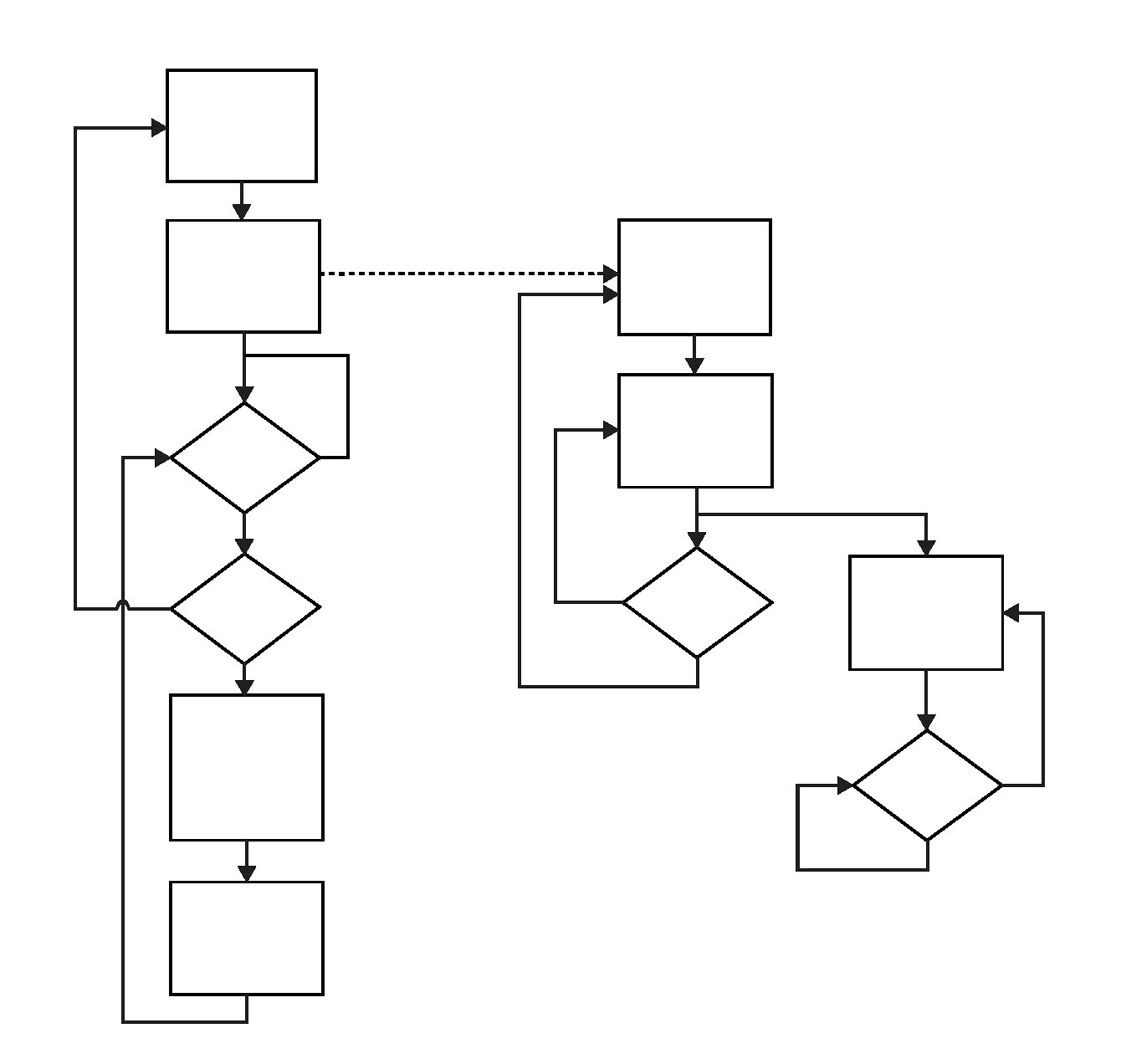This is a detailed black-and-white drawing resembling a complex chart. The illustration uses various geometric shapes, including rectangular boxes and diamond shapes, interconnected by arrows. Positioned on the left side of the image, there are two main rectangular boxes. From the first box, an arrow points straight down, while another arrow emerges and proceeds horizontally. Following this progression, there are alternating diamond shapes and arrows leading to more rectangles and diamonds, creating a structured flow.

Notably, from the second box in the first column, a dashed arrow branches out to the right, connecting to additional boxes. This section contains two rectangles followed by a diamond shape, and in a parallel column, another sequence of a rectangular box followed by a diamond shape is visible. Each shape is interlinked with the others through arrows, illustrating a dependency that resembles a family tree or a brainstorming flowchart.

This interconnected network of arrows and shapes underscores a system where each component is crucial for the entire structure’s functionality, symbolizing the interconnected and contingent nature of the elements. The overall design suggests a cyclical process, reminiscent of the "circle of life," where each part reflects and relies on one another to operate harmoniously.